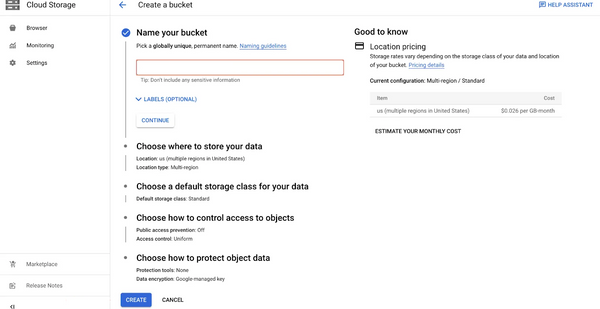The image displays a cloud storage interface with a sleek, white background. In the top left corner, there is a cloud storage logo followed by the title "Cloud Storage." Below this title, a series of tabs are aligned vertically on the left side of the screen, including options for "Browser," "Monitoring," and "Settings." There is a notable gap of white space before three additional tabs appear at the bottom left: "Marketplace," what seems to be "Release Notes," and an indistinguishable tab. The bottom left corner also features a single icon. 

On the right side, the top section prominently features the text "Create Bucket" centered on the screen, along with a prompting line "Name your bucket," accompanied by an input box for user data. The interface further provides sections for choosing data storage location, selecting a default storage class, managing access controls, and protecting object data. In the upper right corner, a "Good to know" information box is displayed. Adjacent to this, there is a blue-colored Help Assistant button, offering additional user support.